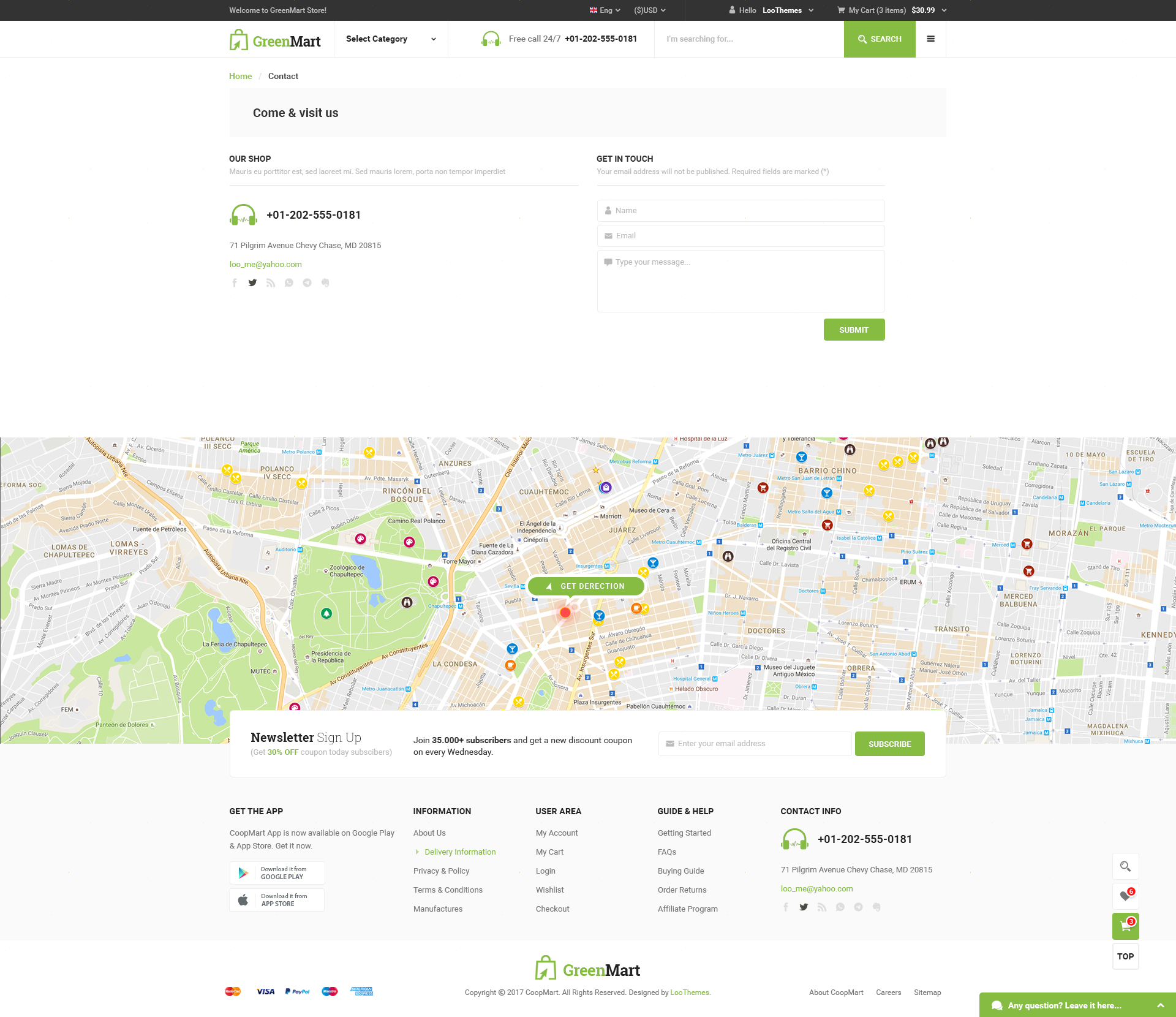The central portion of the webpage prominently displays the map for a company. At the top, a dark black bezel features the greeting "Welcome to Green Market Store" in white text. On the right-hand side, a British flag icon in white with red bands reads "ENG" for English, indicating the selected language, along with a drop-down arrow. Adjacent to it, a dollar sign next to "USD" and a drop-down arrow denote the selected currency, all in gray. A silhouette icon representing a person, comprising a circle for the head and a half-circle for the torso, is labeled "Hello" in gray text. 

To the right, "LOO Themes" appears in bold white with a drop-down arrow, followed by a shopping cart icon also in bold white. Next to the cart, "My Cart" is displayed in gray with "(3 items)" in parentheses. Outside the parentheses, the text "$30.99" in bold white indicates the total cost, accompanied by a gray drop-down arrow.

In the center, the Green Mart logo is in a white area. The logo features a bag with a green arrow pointing to it, with "Green" in green text and "Mart" in bold black. To the right, a black "Select Category" text has a matching black drop-down arrow. A pair of green headphones is shown alongside the gray text "Free call 24/7". Below that, "+01-202-5555-0181" appears in bold black.

On the left-hand side near the Green Mart logo, a navigation option is highlighted in green for "Home", immediately followed by a black "Contact" text separated by a backslash. Below, a dark gray rectangle contains bold black text stating "Come and visit us". 

Two sections appear underneath. The left section shows "Our Shop" in bold black, followed by some gray text in a different language. Beneath this, a headset icon displays the phone number again, followed by their email "lou_me@yahoo.com". Above the email, their address, "71 Pilgrim Avenue, Chevy Chase, MD 20815", is listed in black.

In the right-hand section, "Get in Touch" appears in bold black, followed by gray text: "Your email address will not be published. Required fields are marked" and an asterisk in parentheses. This section features name, email, and message fields indicated by corresponding dark gray icons. Finally, a dark blue-green "Submit" button with bold white text is on the far right.

Below all this, a map with various pins is displayed. At the center, an oval button reads "Get Directions" in bold white text with a bold white cursor. The map has a dark green background with a white shadow box surrounding it, showing the company's contact information.